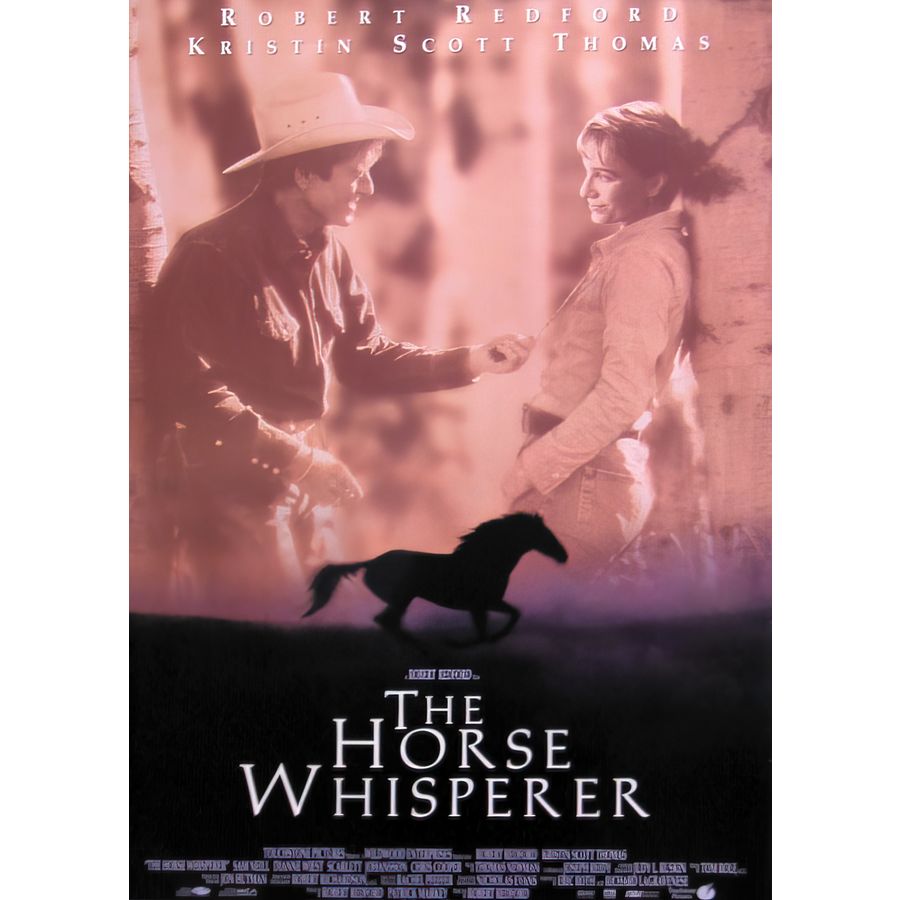This is an advertisement for the film *The Horse Whisperer*. The movie poster prominently features the names Robert Redford and Kristen Scott Thomas in white letters at the top. Both actors are depicted in a sepia-toned background: Redford on the left, wearing a cowboy hat and a cowboy ensemble, and Kristen Scott Thomas on the right, leaning against a tree. Redford appears to be smiling and pointing something at Thomas, who is looking down at him with a subtle smile. Between them and below, there is a horse, linking their visual narrative to the film's theme. The film's title, "The Horse Whisperer," is displayed in bold white capital letters on a black background, with traditional movie credits and the Touchstone Pictures logo beneath, rendered in a less readable, blocked text. Overall, the poster captures a rustic and intimate atmosphere, amplified by the sepia tones and the contrasting black lower section.